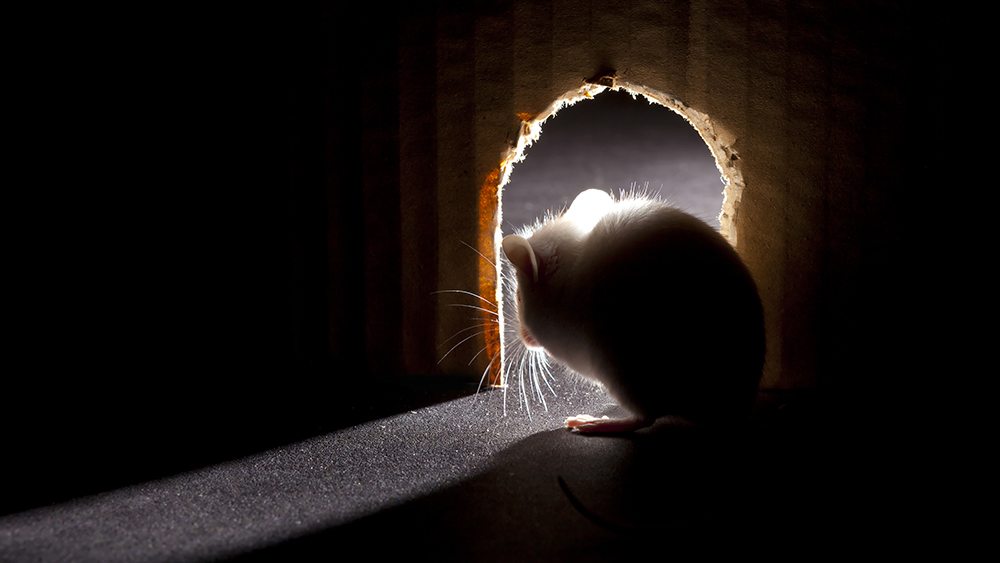This dramatic and otherworldly photograph features a small mouse peering out of a traditional arched mouse hole set against a pitch-black background. The mouse hole, resembling an archway, is cut purposefully into what appears to be a cardboard wall, with subtle light seeping through the material, giving it a soft glow. The mouse, mostly cloaked in shadow, has its white fur illuminated by a light shining through the archway. Positioned at the entrance of the hole, the mouse looks outward with its back to the camera, its head on the left side of the archway and its body on the right. The ground below appears dusty and unclean, contrasting with the smooth, black floor that spreads evenly across the scene. The subtle reflections on the mouse's whiskers add a delicate touch to this mysterious, almost cosmic image.